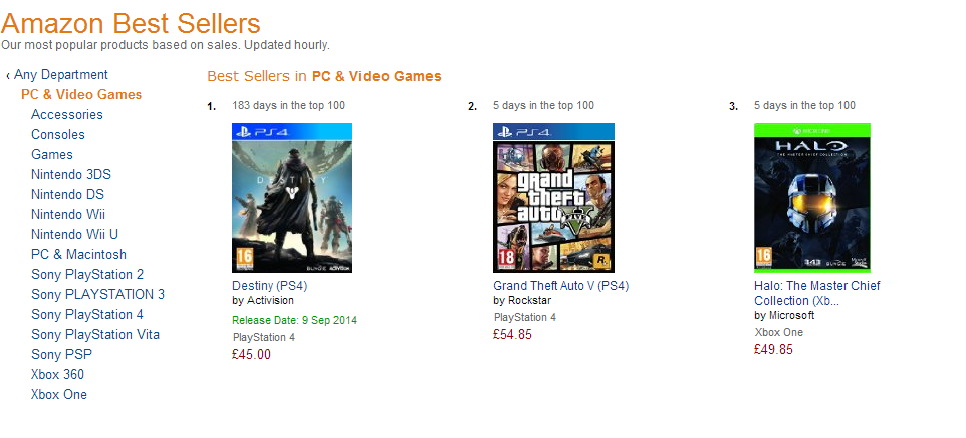The image depicts an Amazon search results page, specifically showcasing the "Amazon Best Sellers" section for PC and video games. The orientation appears to be landscape, and the interface lacks defined borders. 

At the top, against a clean white background, there's an orange header labeled "Amazon Best Sellers," followed by a black subheader stating, "Our most popular products based on sales. Updated hourly." Below this, there’s a navigation interface with a back button labeled "Any Department." A series of selectable links follow this button, with the first option, "PC & Video Games," highlighted in orange to indicate it is currently selected. Additional options listed below include "Accessories," "Consoles," "Games," as well as various Nintendo, PlayStation, and Xbox categories.

To the right, the text "Best Sellers in PC & Video Games" is prominently displayed, with "PC & Video Games" in bold. The first listed best seller is "Destiny" by Activision for 45 euros, noted for being in the top 100 for 183 days, and accompanied by an image of the game. Below that, the second item is "Grand Theft Auto V" for the PS4 by Rockstar, priced at 54.85 pounds. The third listing is "Halo: The Master Chief Collection" for Xbox One by Microsoft, priced at 48.85 pounds. Each of these entries includes their respective cover images.